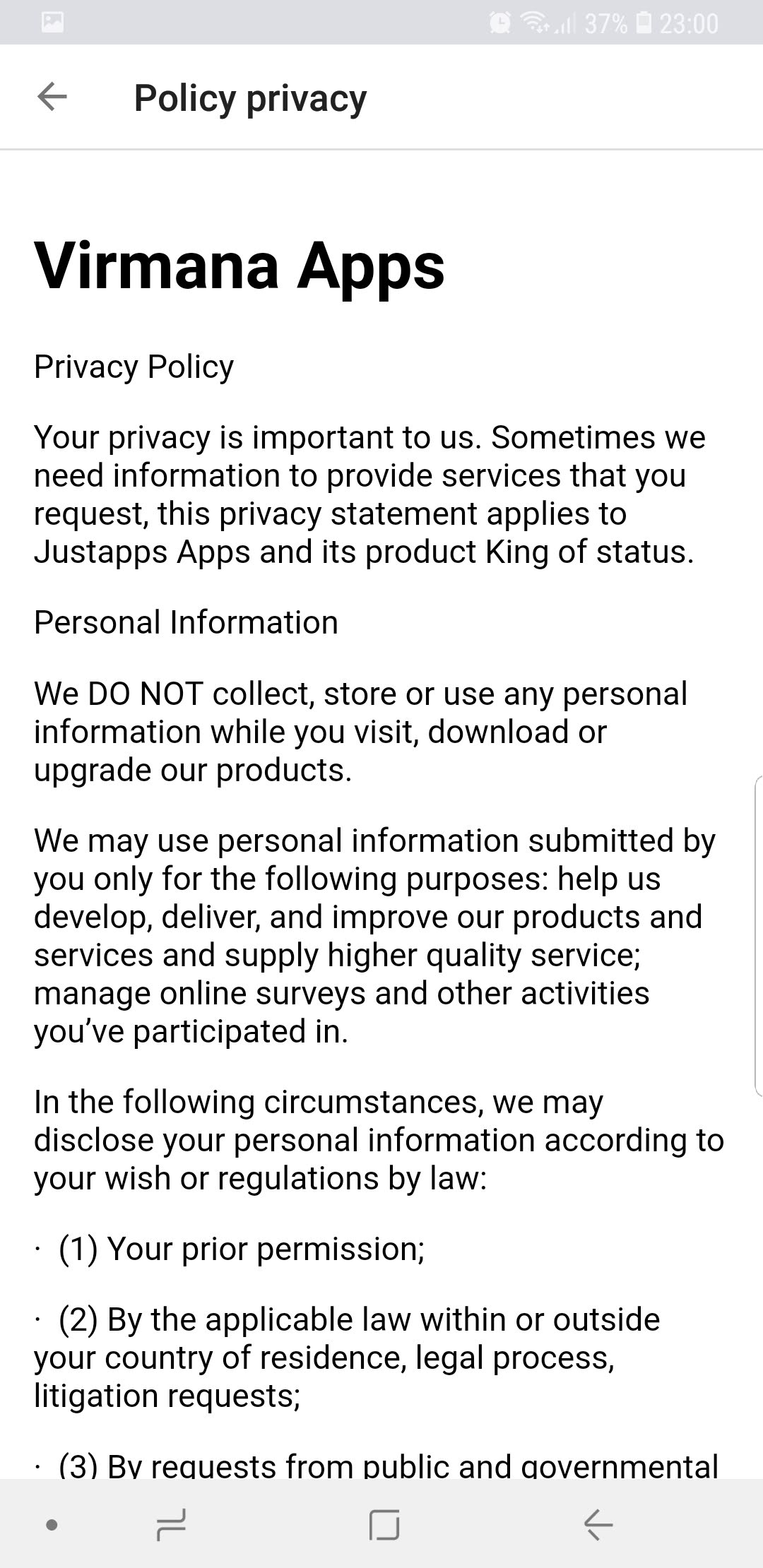The screenshot displays the Privacy Policy section of Vermont Apps. At the very top, the status bar shows the Chrome browser with a clock indicating a time of 23:00 and a battery level of 37%. Below the browser bar, a back button and the title "Privacy Policy" are prominently displayed. 

The header reads "Privacy Policy" in larger, bold black letters and is followed by "Vermont Apps." Beneath this, the policy begins with a statement that highlights the importance of user privacy, stating: "Your privacy is important to us. Sometimes we need information to provide services that you request. This privacy statement applies to just apps and its product king of status."

Following this introduction, there is a section titled "Personal Information," which contains several paragraphs. It reassures users that no personal information is collected, stored, or used while they visit, download, or upgrade Vermont Apps' products. The policy further explains that personal information submitted by users may be used for specific purposes such as helping to develop, deliver, and improve products, providing services, and managing online services.

Additionally, the policy outlines scenarios in which personal information may be disclosed, including:
1. With the user's prior permission.
2. In accordance with applicable laws, whether within or outside the user's country of residence, due to legal processes or litigation requests.
3. Upon request from public and governmental authorities.

The bottom of the screenshot features icons for phone-related actions, marking the end of the policy text.